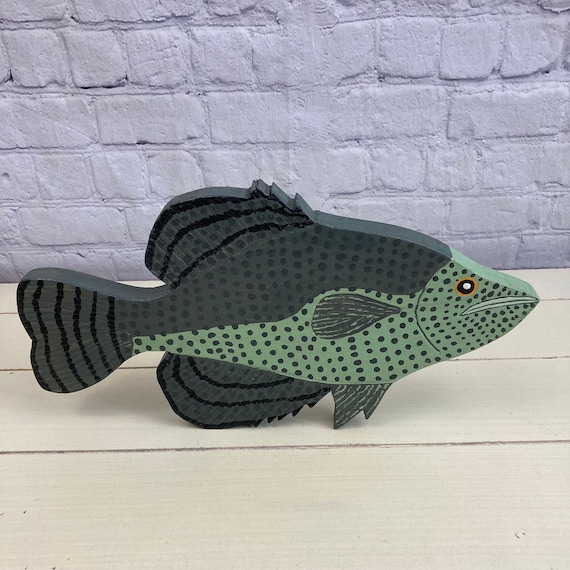In the image, there is a finely crafted wooden fish carving positioned prominently in the middle of a light wooden table. The table is situated in front of a pastel purple painted brick wall, serving as the backdrop. The fish itself is detailed with a blend of colors: the top is a blend of light bluish-gray and dark green, transitioning into a lighter green towards the bottom. Its body is adorned with dark grey and black polka dots. Notable features include black stripes on the top and bottom fins, which have a distinctive black border, and vertical black stripes on the tail fin. An intricate black circle eye with a yellow ring around it stands out. The fish appears to be painted with care, capturing the essence of a real fish, and is oriented to the right. The overall scene showcases the craftsmanship of the wood carving against a quaint, pastel-colored setting.